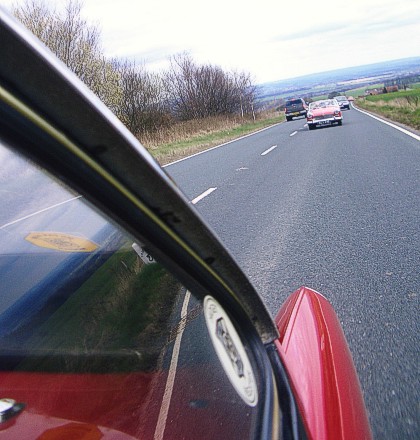In this image, captured from the passenger's perspective, we observe a vivid urban scene through the window of a red car. The car’s black window frame prominently features in the photo’s edge. The two-lane road ahead is depicted in shades of gray with white dashed lines demarcating the lanes. Dominating the scene is the front view of a pink car directly ahead, followed by another vehicle behind it. To the left, there's a partial view of the rear side of a gray car. The surroundings feature leafless trees on the left, with patches of green grass below them. On the right, more green grass can be seen stretching into the distance. The horizon reveals an expansive view leading to a sky that appears white, interspersed with a few narrow, gray clouds.